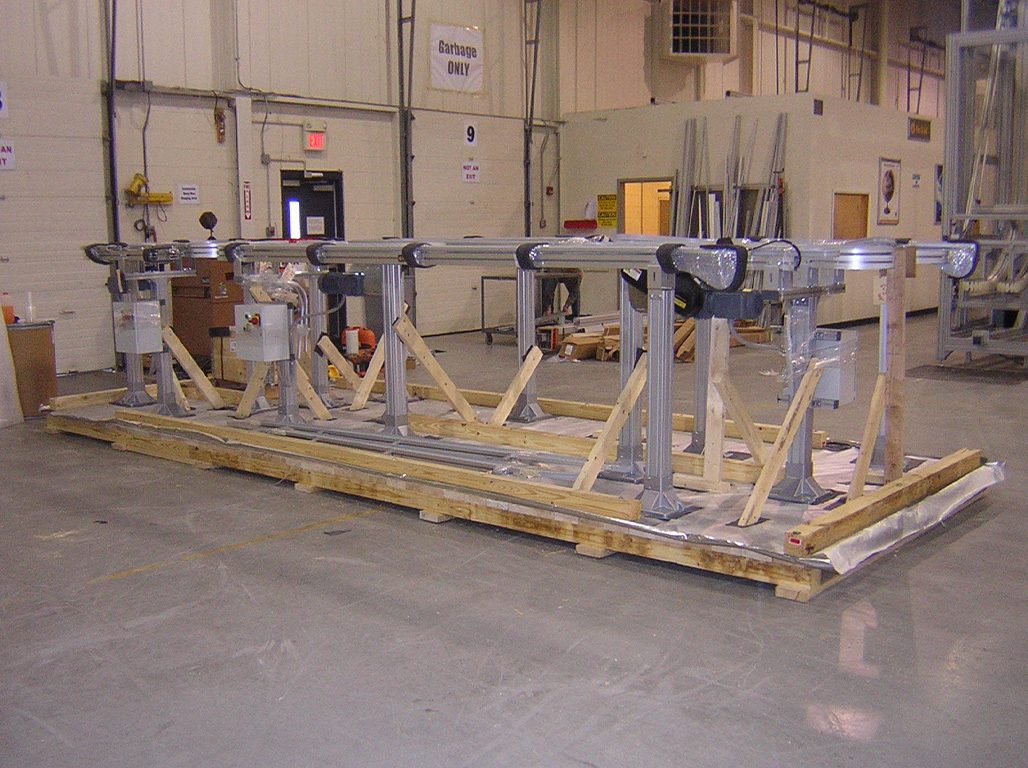Inside a spacious factory with a concrete floor, the photograph captures a large piece of machinery in the foreground, meticulously prepared for shipment. The machinery, composed of interconnected metal components, is meticulously secured with cellophane, ensuring stability during transit. It rests on a massive pallet constructed from wooden 2x4s, and a winding conveyor belt runs across its length, indicating its industrial purpose. Adjacent to this setup is a loading dock area, flanked by walls made of brick and metal, all painted in an off-white hue. Various signs adorn these walls, including a "Garbage Only" notice, a large number "9," and a "Not an Exit" sign above a warehouse door that slides up. An illuminated red exit sign hangs above a black door to the left. Toward the back right of the image, a protruding office space with two white doors overlooks the loading dock. The factory appears devoid of people, emphasizing the orderly and methodical arrangement of the workspace.